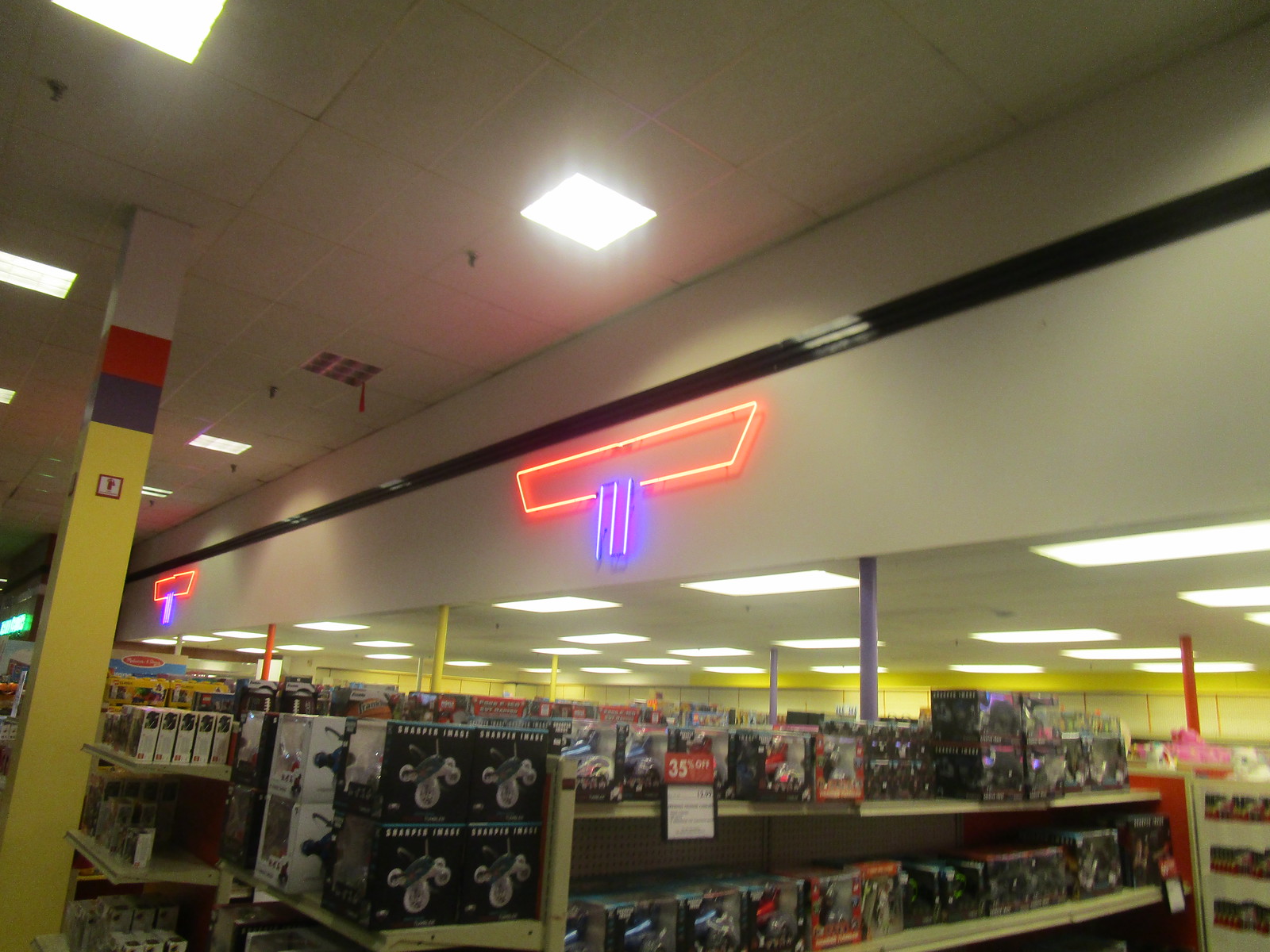The image depicts a vibrant retail store interior characterized by its colorful decor. The walls are painted a bright yellow, and a distinctive square post near the center of the store features bold yellow, blue, and red bands. Neon signs add to the lively atmosphere, with an orangey-pink parallelogram design and vertical neon purple lines. Above, the ceiling is outfitted with standard drop tiles and fluorescent lighting. The store's shelves are neatly organized with numerous boxes of goods, though the specific products are indiscernible from the image. A prominent red sign advertising a "35% off" sale is visible on the closest shelf. The scene is noticeably devoid of any customers or staff.